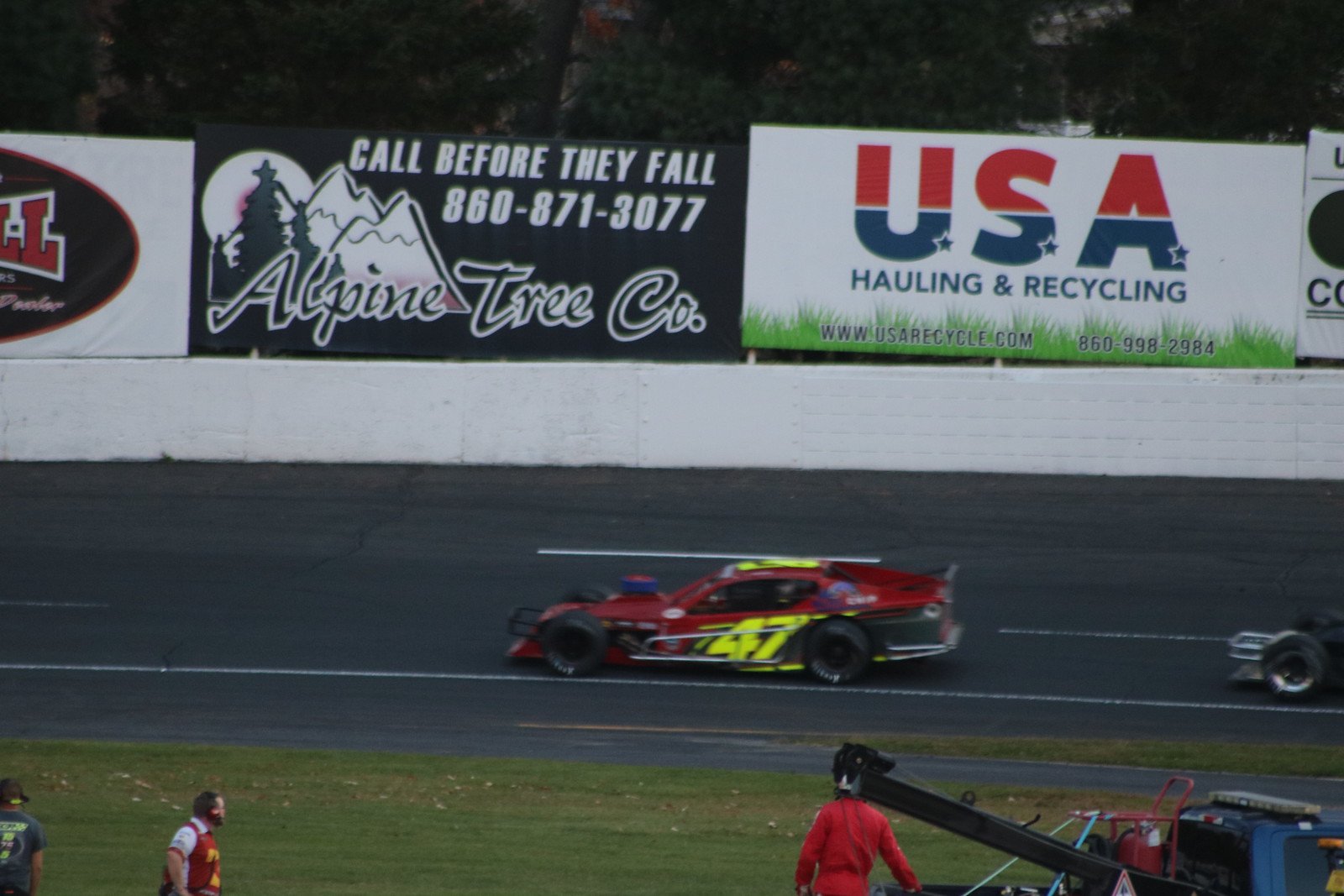The image captures an outdoor stock car racing event on a gray asphalt track surrounded by various advertisements. Dominating the center is a red and black car with a highlighter yellow number 47 prominently displayed on its side and top. Another car, of which only the front tires are visible, seems to be trailing behind. The barricade around the track features several advertisements, including a black-and-white ad for Alpine Tree Company with the slogan "Call Before They Fall" and a logo depicting mountains and the moon, and another ad for USA Hauling and Recycling with red and blue lettering. In the background, a dense collection of trees frames the scene, while in the foreground, green grass is visible. Three men are near a tow truck, one dressed in red, standing by the track. The photograph, taken during the day, also captures a crowd watching the race from a field beyond the barricades.